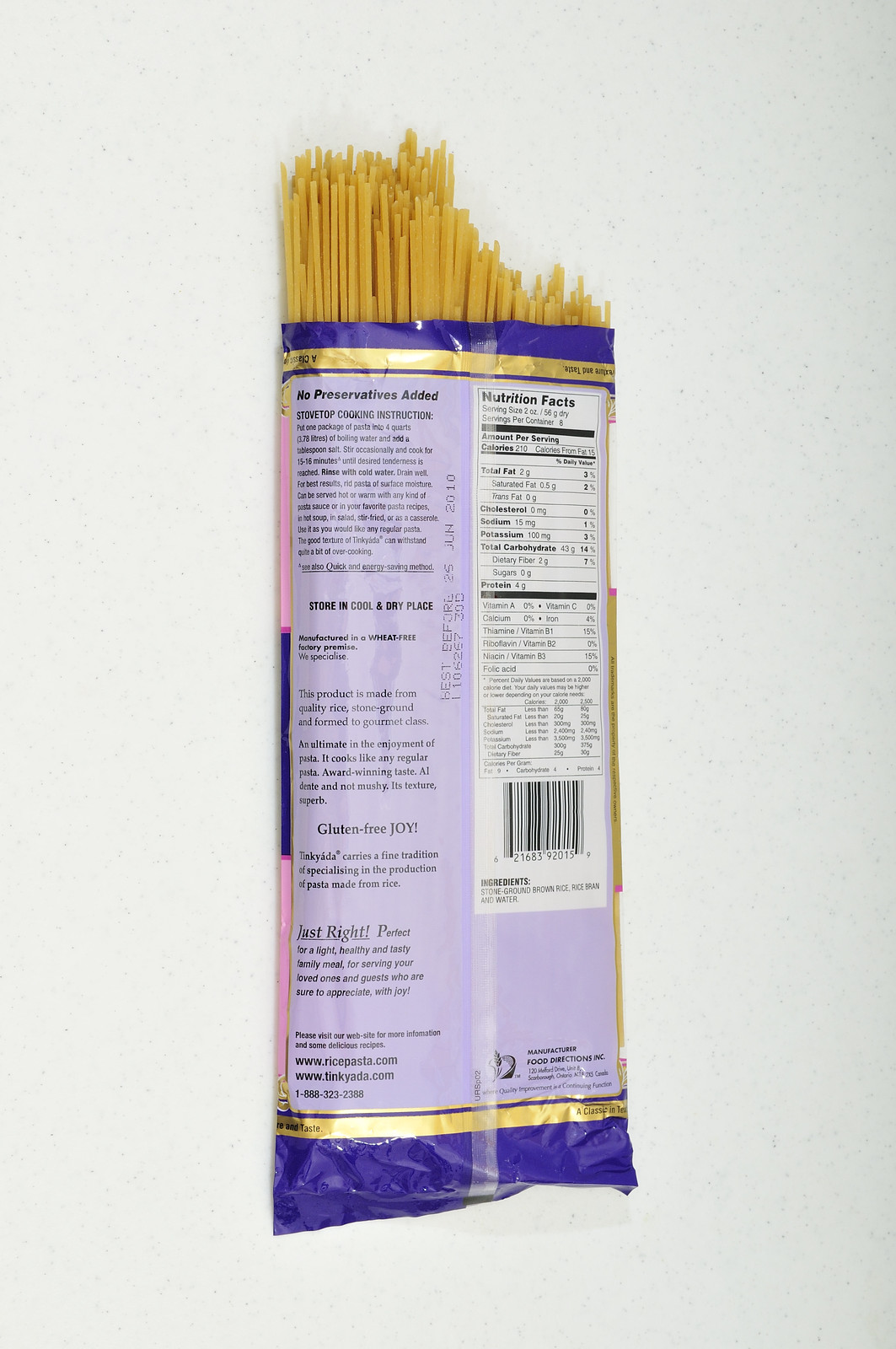This image shows the back of a bag of gluten-free spaghetti pasta, made of straight, long noodles with some sticking out of the opened top. The background is white, highlighting the detailed packaging. The bag is predominantly purple, with notable color bands: a purple band at the very top, followed by a gold band, and a dark blue band at the bottom. The top blue band carries a notice of "No preservatives added" and stovetop cooking instructions, while the gold band beneath it adds to the decorative look. 

The central area of the bag features extensive product information. On the right side is a large white rectangle containing nutritional facts in black lettering, which occupies about two-thirds of the bag. Below the nutritional information, there is a QR code. Additionally, the bag advises consumers to store the product in a cool, dry place and notes that the best-before date is June 26, 2010. The left side has more comprehensive details, including cooking instructions and information about the product being gluten-free. The web address, "www.ricepasta.com," is printed on the bag, and there seems to be a mention of the product being made from quality ingredients, although it’s hard to read. The presence of some pink accents on the front adds a subtle touch of color to the packaging.